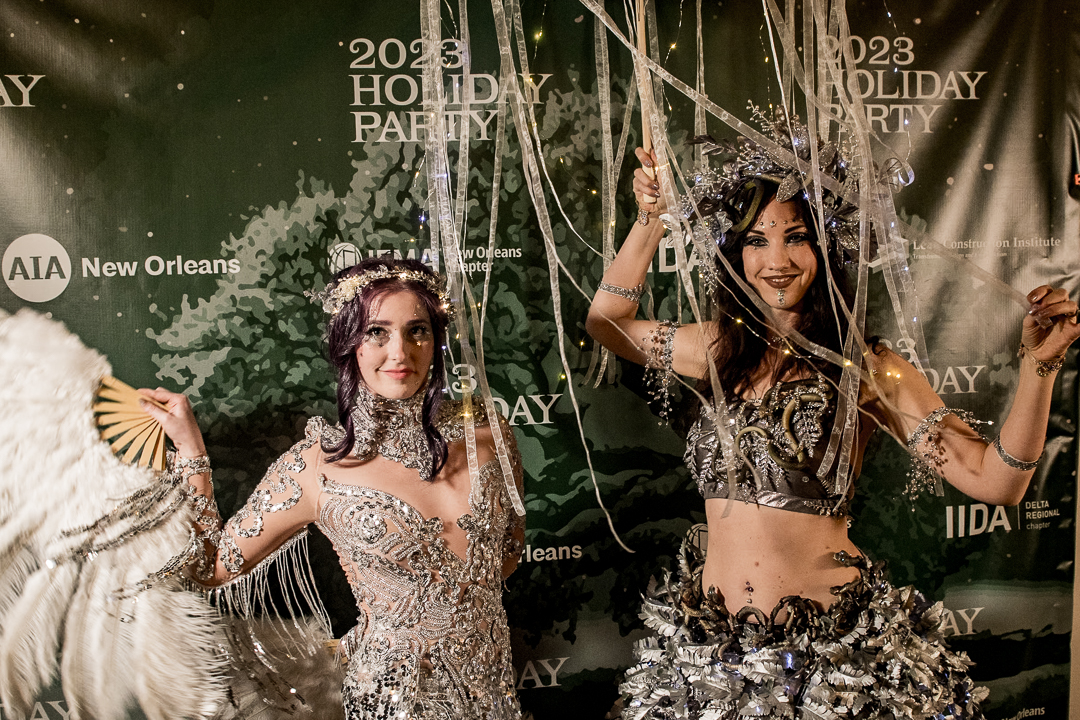The image depicts two women at a lively 2023 Holiday Party for AIA New Orleans and IIDA Delta Regional, as indicated by a prominent backdrop. They are dressed in elaborate, stage-like costumes adorned with intricate beadwork, sequins, and numerous accessories, including tiaras, bracelets, and armbands. The predominantly silver outfits feature elements of black and white, with one woman sporting a midriff top and leaf-patterned bottom, evoking a Medusa-like appearance. Both women have decorated hair, embellished with light-up garland and festive ornaments. One woman holds a large feather fan, while the other has tinsel streamers. They're clearly enjoying the celebration, smiling under vibrant makeup and shimmering with glitter, fully embodying the festive spirit of the event.